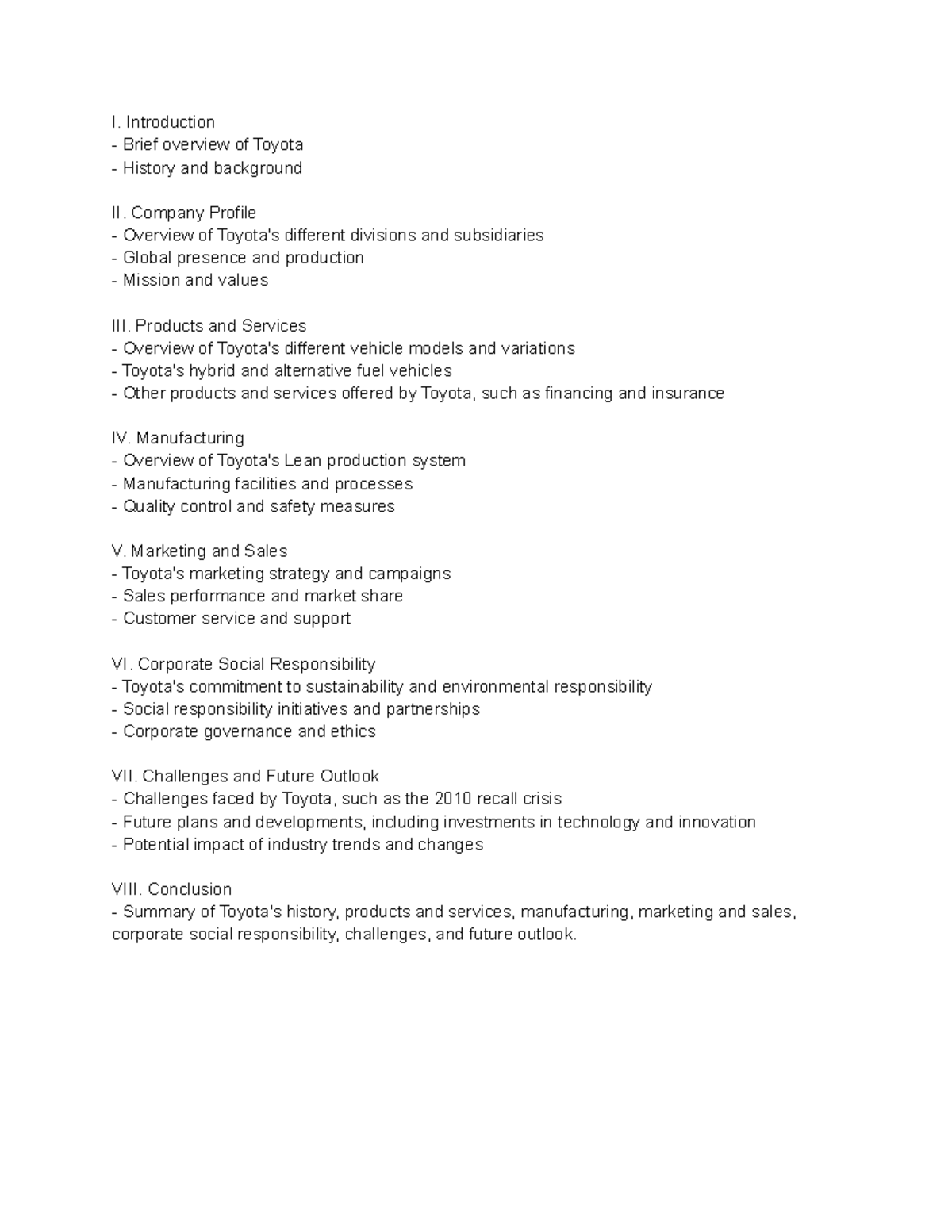This image depicts a low-resolution, text-heavy outline for a detailed presentation on the Toyota Corporation, displayed on a white background with black text. The content is organized using Roman numerals to separate each major section, with two to three succinct bullet points beneath each item, summarizing the key topics to be covered. The sections include:

I. Introduction
   - Overview
   - History and Background

II. Company Profile
   - Company Structure
   - Key Executives
   - Financial Performance

III. Products and Services
   - Vehicle Models
   - Technological Innovations
   - After-Sales Services

IV. Manufacturing
   - Production Processes
   - Global Manufacturing Plants
   - Quality Control

V. Marketing and Sales
   - Market Strategies
   - Sales Performance
   - Customer Engagement

VI. Corporate Social Responsibility
   - Sustainability Initiatives
   - Environmental Responsibility
   - Social Initiatives and Partnerships

VII. Challenges and Future Outlook
   - Industry Challenges
   - Strategic Goals
   - Innovation and Growth

VIII. Conclusion
   - Summary of Key Points
   - Future Outlook

Each bullet point is brief, typically five to ten words, making it a clear and effective outline for guiding a speech, presentation, or essay. The Conclusion section stands out as it uses a dash instead of bullet points, indicating a need to summarize the entire presentation and mention Toyota's future prospects. The overall layout is clean and concise, making it a practical tool for structuring comprehensive content about the Toyota Corporation.